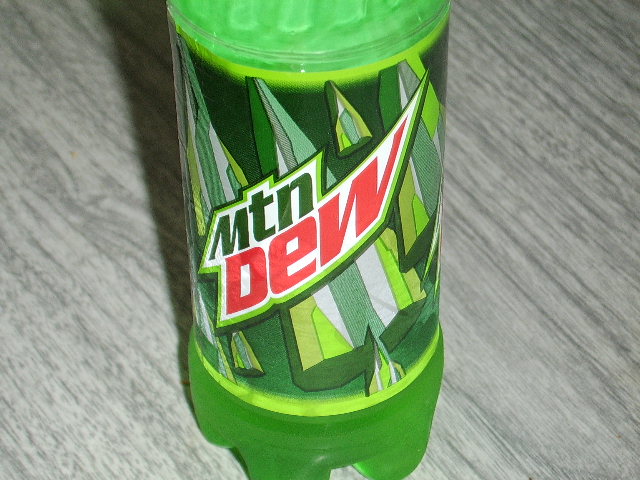This photograph features a small bottle of Mountain Dew, showcasing approximately 75% of the bottle with the lid out of the frame. The iconic Mountain Dew logo is prominently displayed in the center of the label, slanting upwards from left to right. The label features "MTN" written in dark green lettering and "DEW" in red lettering against a white background. Surrounding this text is a dynamic green background designed to mimic mountainous terrain, with spiky, triangular shapes in varying shades of green and white. The clear bottle itself contains the vibrant green soda, with a light foaming visible near the top, suggesting the soda's effervescence. The bottle is resting on a gray wood grain countertop or table, adding a rustic touch to the image's setting.